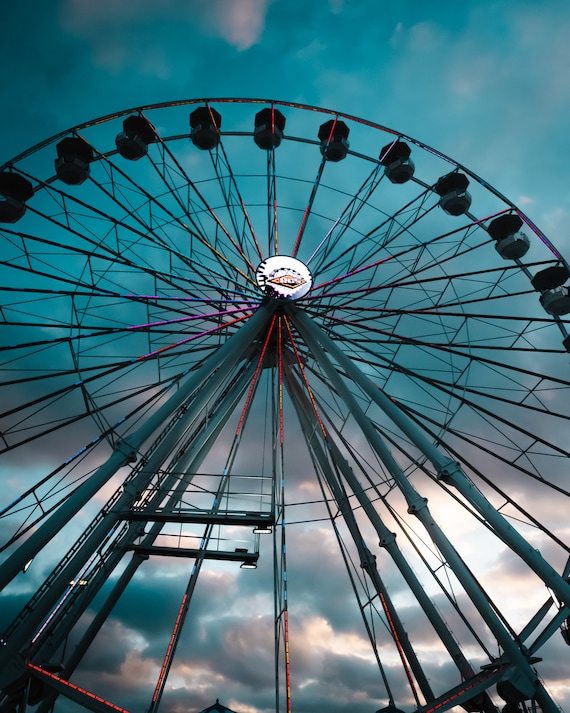This vertical photograph captures the grandeur of a towering Ferris wheel from a ground-up perspective. The massive wheel features basket gondola seats designed to give riders a scenic loop around. At its center, an illuminated white sign hosts a red diamond with unreadable white text, hinting at some form of branding or naming. The structural frame and spokes of the Ferris wheel are a mix of dark gray and red, adding to its striking appearance. The sky above is ominous with dark, brooding clouds, accentuated by the pink-tinged cloud tops, suggesting that the photograph was taken around sunset or early twilight. The image conveys a dramatic juxtaposition of the vibrant Ferris wheel against the foreboding sky.